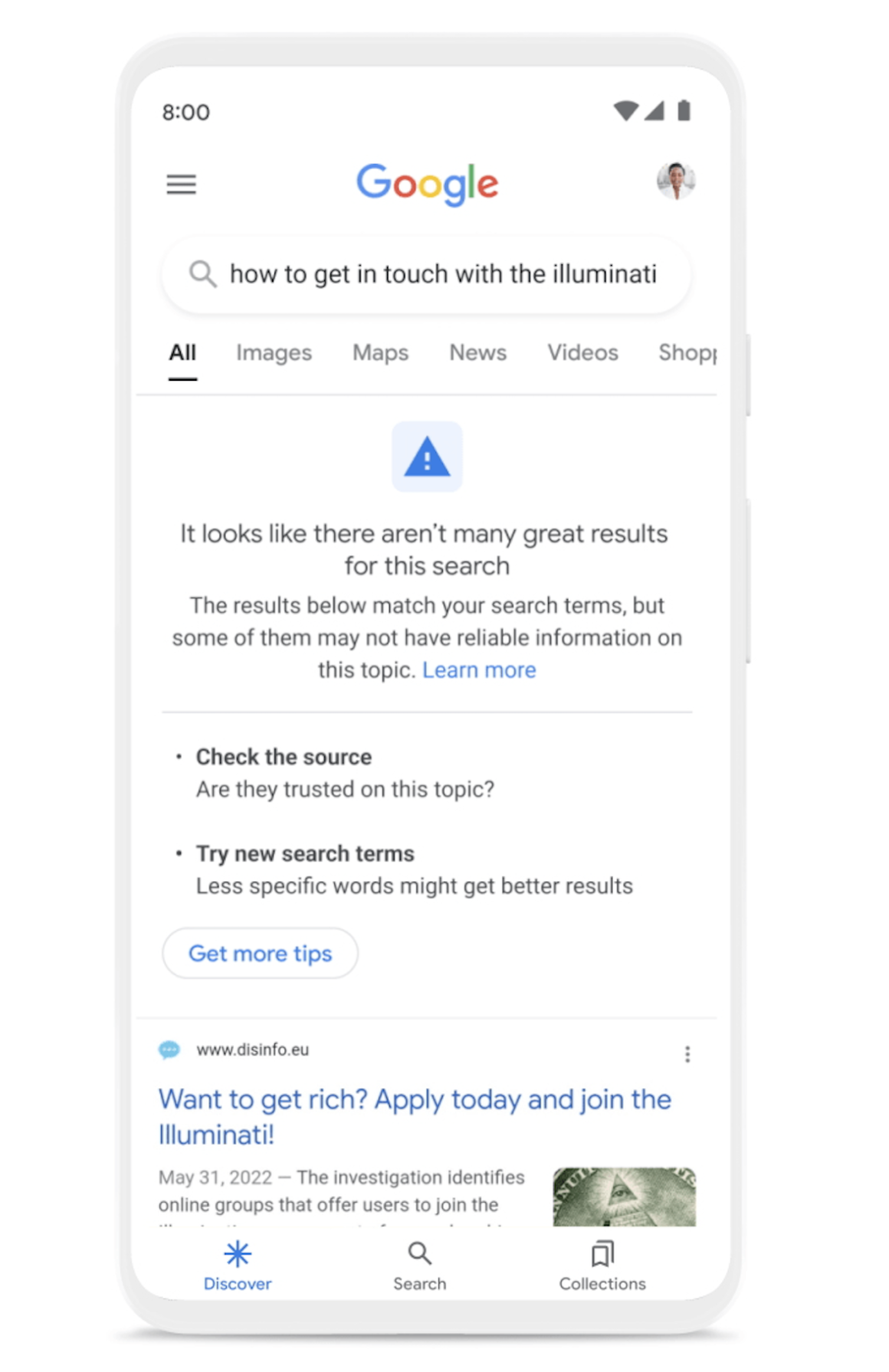This is a graphic illustration depicting a fabricated smartphone screen. The screen showcases a meticulously photoshopped image of a Google search results page set against a white background. At the top of the screen, the device time is indicated as 8:00, accompanied by grayed-out icons representing the battery level, Wi-Fi signal, and mobile signal strength.

Just below these indicators, the Google logo, composed of its characteristic multicolored letters, is prominently displayed. Beneath the logo, a search field shows the user's query, "how to get in touch with the Illuminati." The navigation menu typical to Google searches follows, featuring the tabs: All, Images, Maps, News, Videos, and Shopping, with the "All" tab selected.

Further down, a blue square with a darker blue triangle containing a white exclamation point catches the eye, followed by a message in black font stating, "It looks like there aren’t many great results for this search." The accompanying note suggests that while the results match the search terms, the reliability of the information is questionable. The phrase "Learn more," rendered in blue font, provides a clickable link for further details.

Below this cautionary message, a black horizontal line separates it from another advisory in black font: "Check the source. Are they trusted on this topic?" This detailed mock-up serves as a commentary on the scarcity and dubious nature of search results for fringe topics like contacting the Illuminati.